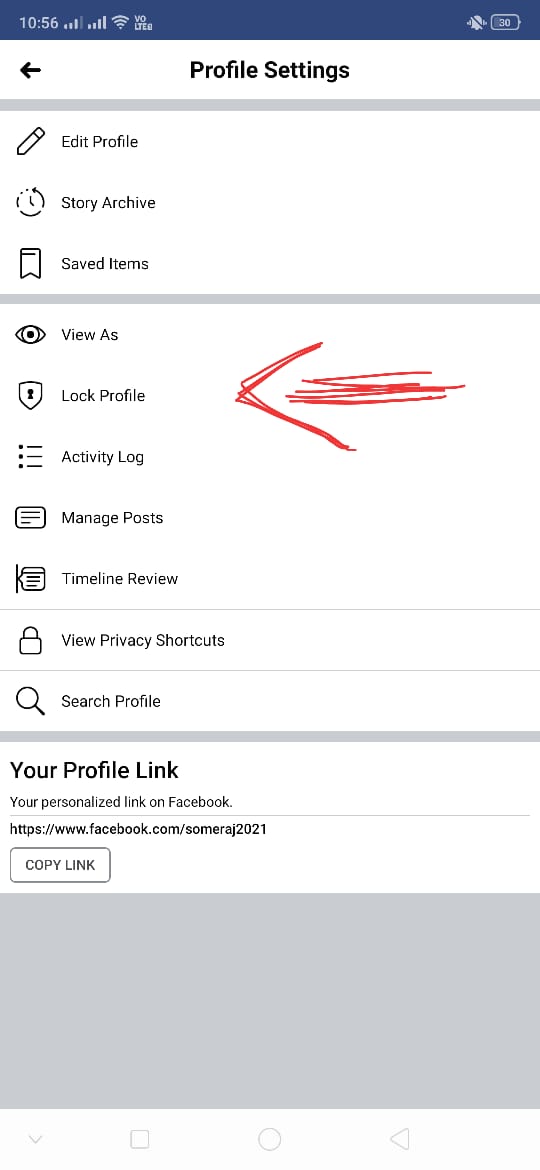The screenshot depicts a detailed view of the "Profile Settings" page on a mobile device. At the top, a blue bar displays the time "10:56" in white text, alongside two signal bars, a white line, the "3G" indicator, and the battery icon.

Beneath the blue bar, the screen transitions into a white area where "Profile Settings" is prominently written in black, accompanied by a left-pointing arrow. Below this section is a separating gray line.

The next segment shows an option titled "Edit Profile" with a pencil icon. Following this are options labeled "Story Archive" with a clock icon and "Saved Items." Under these options sits another gray line. 

Further down, there is a "View As" option adorned with an eye icon and "Lock Profile" which is signified by a shield bearing a key lock symbol. Underneath "Lock Profile," an arrow is hand-drawn to emphasize this feature.

The screen also includes options for "Activity Log", symbolized by three bars, "Manage Posts" with a post square icon, and "Timeline Review" with its respective icon. 

Towards the bottom lies a search bar followed by another gray line. Below this, it states "Your Profile Link: Your personal link on Facebook," providing a web address for the profile that can be copied. Finally, a large rectangle with a gray bottom section is visible at the page's end.